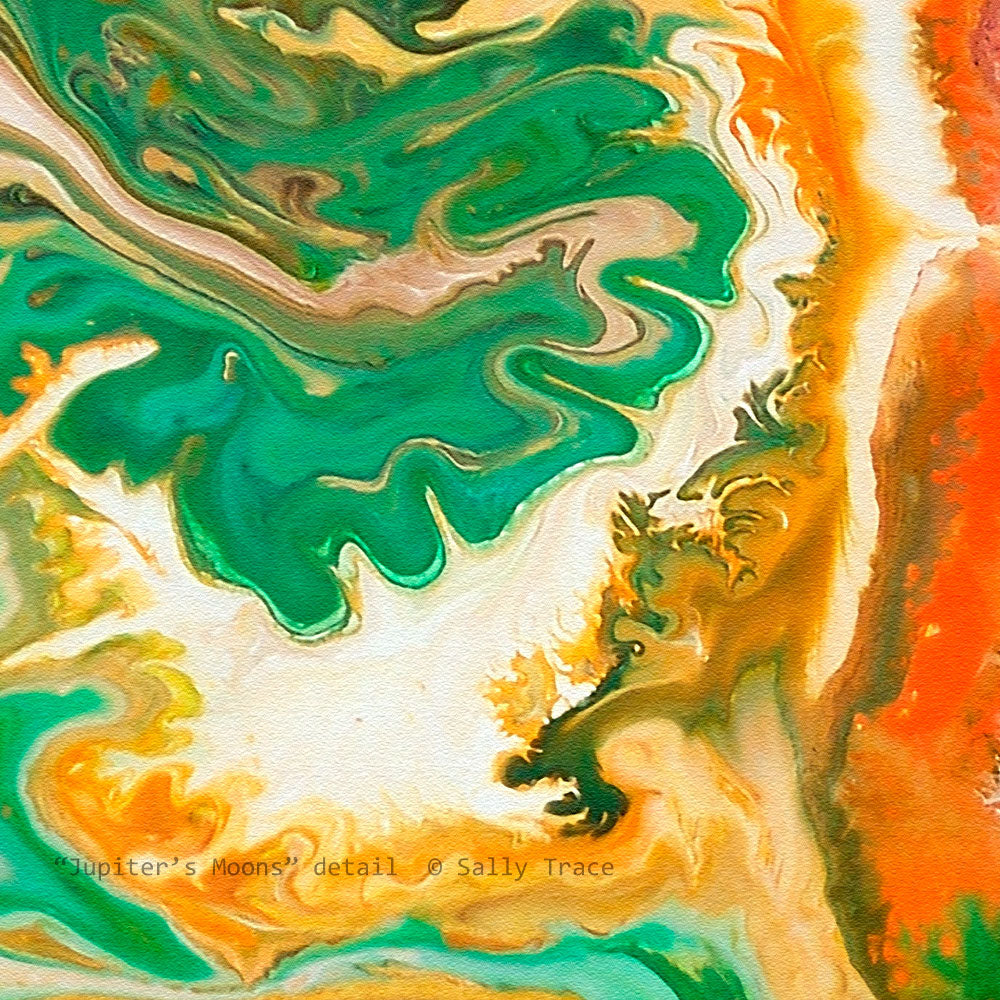This abstract artwork, titled "Jupiter's Moons, Detail," by Sally Trace, is a vividly colored, square piece featuring jagged, fiery orange and green paints. Approximately 30-40% of the artwork is dominated by green, interspersed with around 20% orange, creating a dynamically textured surface reminiscent of a high aerial view of a lake with numerous coves, small peninsulas, and intricate water bodies. The top left corner showcases green with wavy brown lines and white spaces underneath, while the middle hosts a patch of fiery orange that drifts towards the bottom right, flanked by wavy green. The right side is characterized by an interplay of orange hues and thin white lines, merging into splotchy patterns. The swirling, patterned design echoes the look of an oil spill, with its fluid, dynamic movement. At the bottom left, the artwork is labeled with the title, "Jupiter's Moons, Detail," and signed "Sally Trace," marking it as a distinct, detailed creation that captures the viewer's imagination.